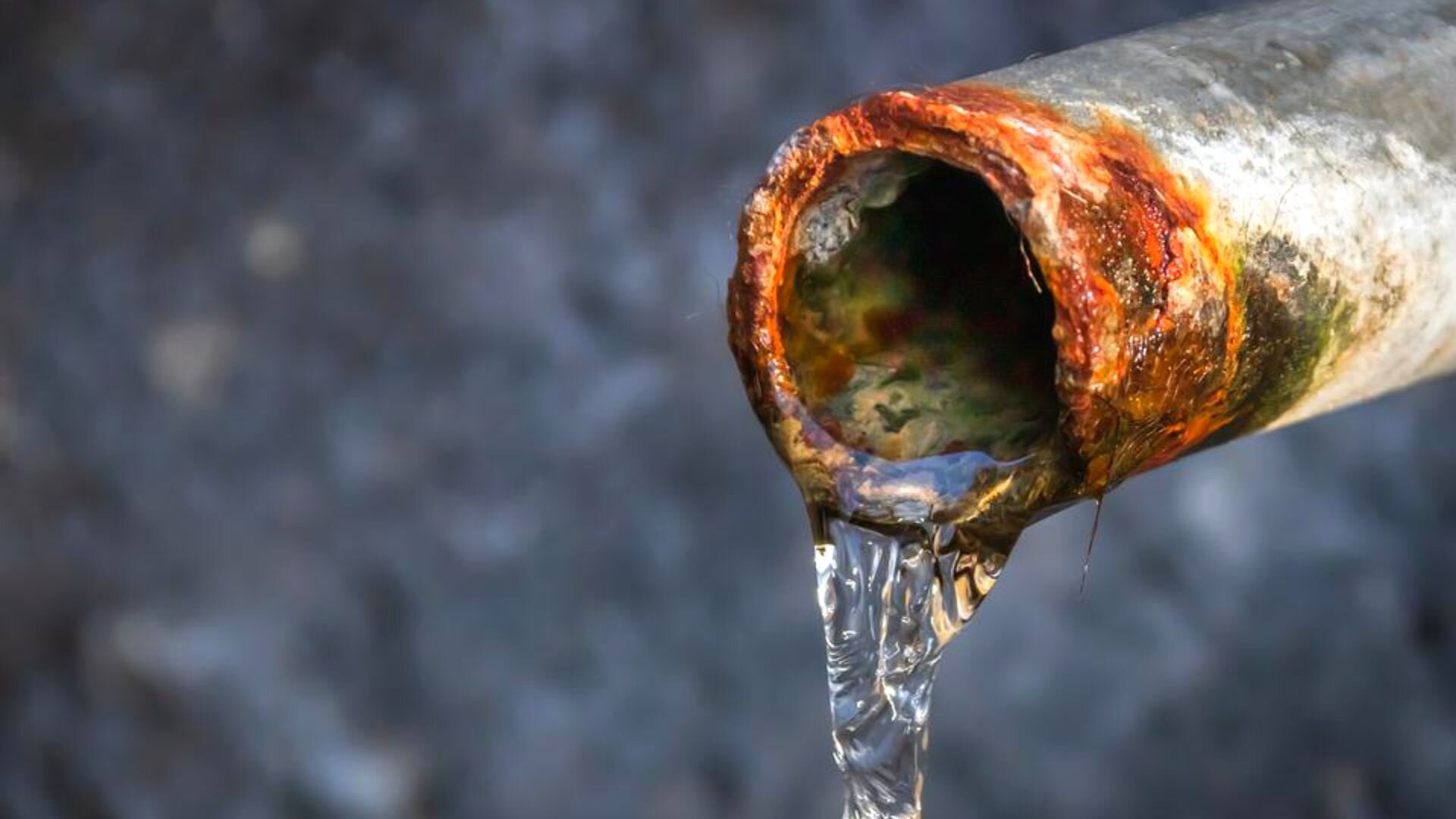The image depicts an aged, corroded metal pipe extending from the upper right corner toward the center, angled downward to the bottom left. The pipe's tip, prominently situated near the center, is heavily oxidized with a rusty orange and brown hue, accompanied by patches of green mossy mold both on its surface and inside. Crystal clear water flows moderately from the pipe, unaffected by the corrosion. The background is heavily blurred, creating a strong bokeh effect that makes it challenging to discern any specific details, though it vaguely resembles either gravel or dirt. This close-up portrait highlights the contrast between the pristine water and the deteriorated state of the pipe.